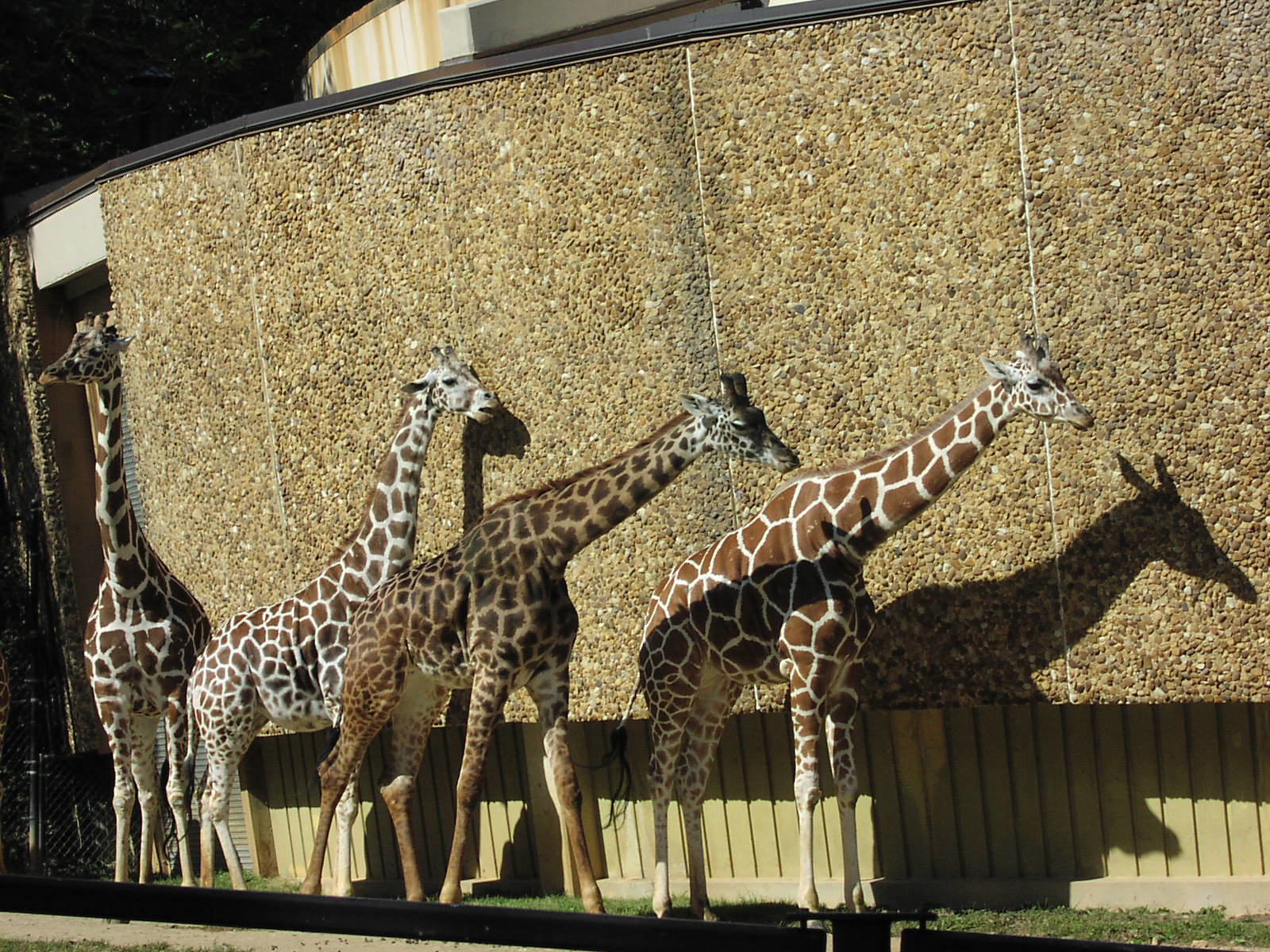In this detailed photo of a zoo, four giraffes are seen lined up in a unique arrangement in front of a tall, beige rock wall with shadows cast prominently behind them. The wall, which appears to be slightly taller than their necks, is brown and rocky with a distinctive gravel texture and brown outlines. The giraffes exhibit varying fur patterns: the first, a brown and white giraffe, stands slightly ahead with its neck inclined down and forward. Behind it, the second giraffe displays darker brown hues, while the third has a lighter, more prominent white pattern. The last giraffe in the lineup extends its neck fully upward, showcasing a dark brown and white pattern. The scene is set against a background that includes some grass, a hint of a beige building, and a black element at the bottom that might suggest a gate or fence. The detailed alignment, position, and shades of the giraffes vividly capture the essence of this moment in the zoo.